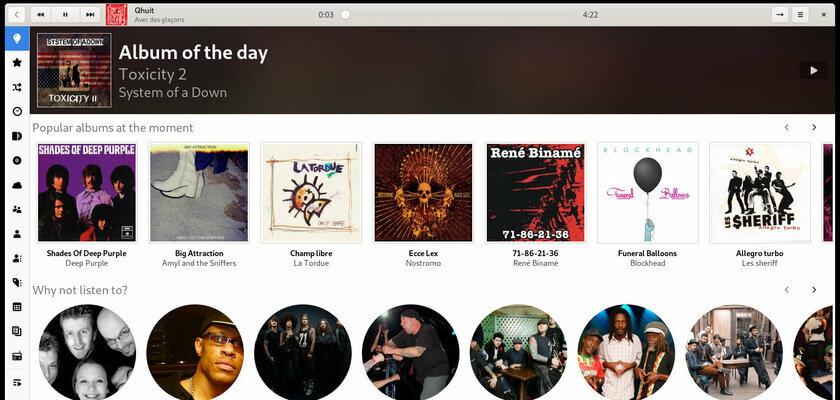The image displays a detailed view of a comprehensive music app interface. At the top, the app highlights a currently playing track by "Q Hewitt" (though the artist's name is noted as uncertain), with playback controls that include options for back, forward, and pause. The track is three seconds into a total duration of four minutes and twenty-two seconds, with the play bar indicating minimal progression. 

Following this, the app features an "Album of the Day" section showcasing "Toxicity 2" by System of a Down, accompanied by its album cover. Below this section, there are seven visible album covers, with additional covers extending off the screen.

Further down, there is a section for artists, represented in circular thumbnails, showing various bands on a blue background. Visible albums include:

1. "Shades of Deep Purple" by Deep Purple
2. "Big Attraction" by Emil and the Sniffers
3. "Champ Libre" by Latour
4. "Echolex" by Nostromo
5. "71-86-21-36" by Rene Benarme
6. "Funeral Balloons" by Blackhead
7. "Allegro Turbo" by Les Sheriff

At the bottom of the screen, under the heading "Why Not Listen To," there are various band images without visible text, suggesting more information might be available if the screen were fully visible.

On the far left, there's a vertical menu with numerous icon-based options, including symbols like a light bulb, a star, a cross blend, and a clock. However, the specific functions of these icons are not immediately clear from this visual representation.